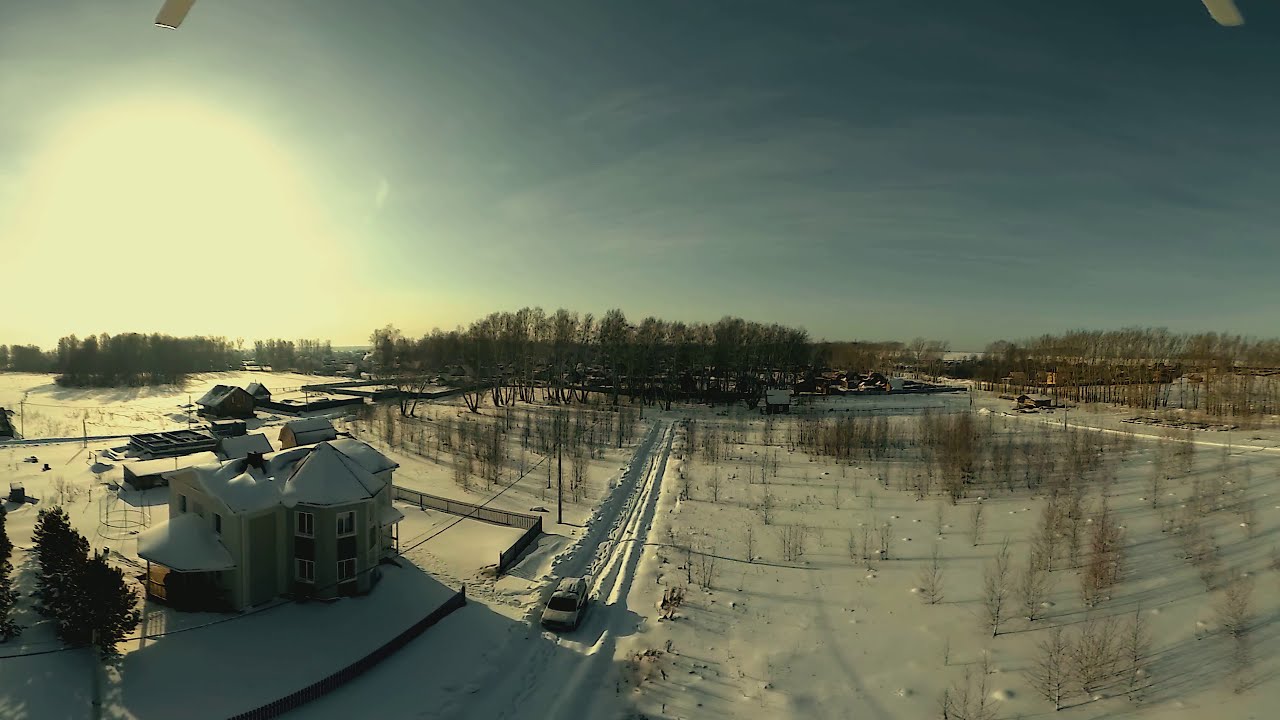An aerial photo captures a snow-covered rural area, showcasing a picturesque winter scene. Taken from an elevated position, the image is slightly blurry but details a landscape blanketed in thick snow. In the foreground to the bottom left, a two-story house with a snow-filled roof and a dome peak stands prominently. The house features multiple windows divided by a white bar, and a black fence encircles its sides while connecting to a smaller, flatter building behind it. Another flattish structure, featuring an opening at the top, is nestled adjacent. Across the snow-plowed road that cuts through the center of the image, another house similar to the first can be seen, accompanied by a smaller house to its right. The road, clear from plowing, reveals the height of the displaced snow and is traveled by a grayish van moving towards the viewer. To the right side of the image, there is a snow-covered field dotted with bare trees devoid of leaves and a few resilient evergreen trees. The backdrop features a tree line under a clear blue sky with a few wispy clouds, adding to the serene and frosty winter atmosphere.